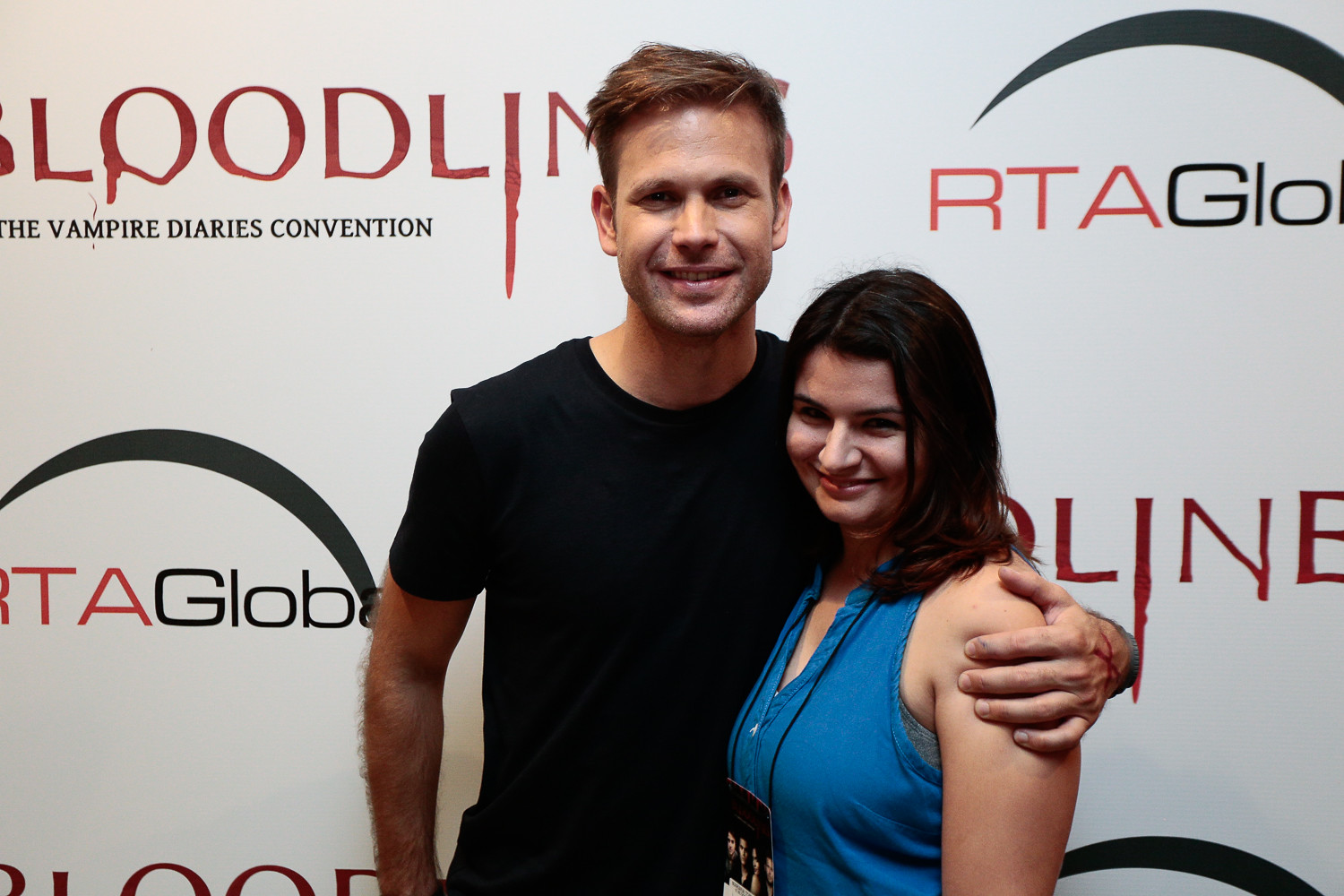The photograph depicts a white Caucasian man and woman attending a red carpet event for the "Bloodline: The Vampire Diaries Convention." The background is a white banner adorned with repeated logos for "Bloodline" featuring red, blood-like dripping text, as well as the "RTA Global" logo with a black swoop. The man, positioned on the left, has brownish-blond hair and is smiling brightly with his mouth open. He is wearing a black t-shirt and has his left arm, marked with a red X, wrapped around the woman. The woman, standing on his right, has shoulder-length brown hair and is dressed in a sleeveless blue top over a gray undershirt. She is wearing a large black lanyard with a pass featuring multiple faces, possibly including the man's. Smiling more bashfully, she faces slightly to the side with her head slightly down. The entire scene is set against the repetitive backdrop of the convention's branding, emphasizing their presence at the event.